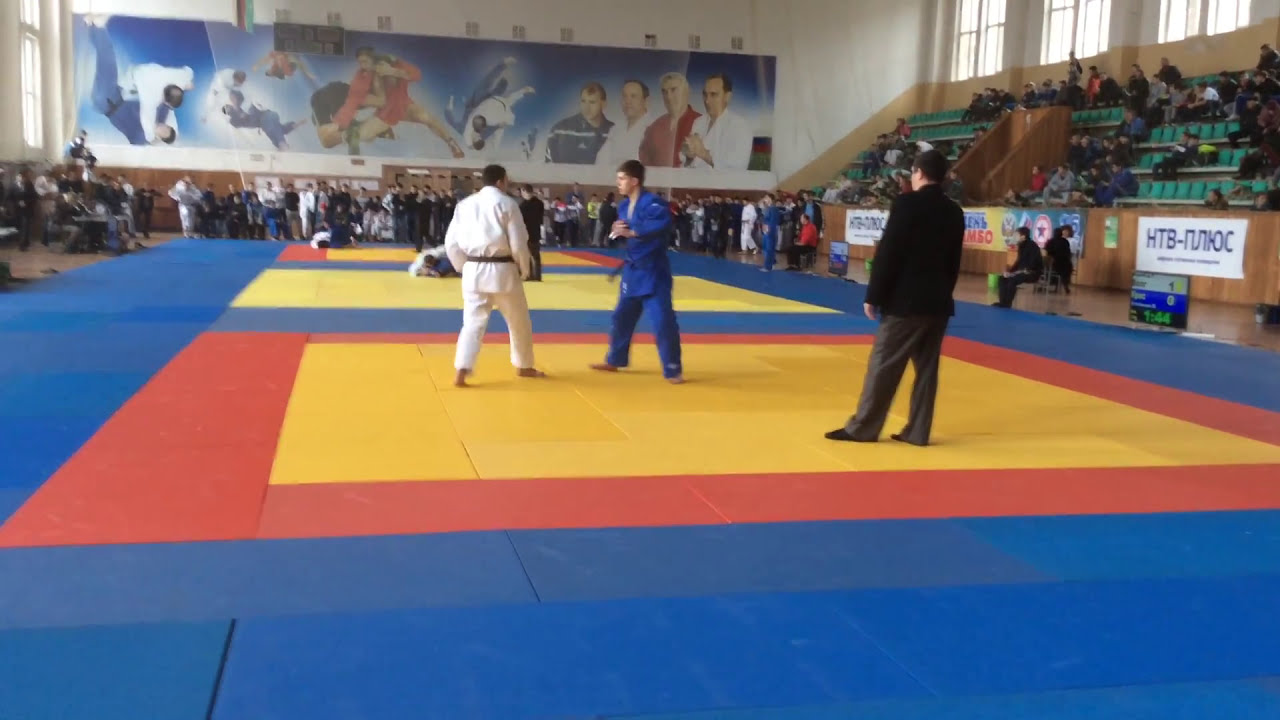Inside a spacious gymnasium, a martial arts competition is taking place with several matches unfolding on alternating mats. Each mat features either a yellow square surrounded by a red border or a plain yellow square. In the forefront, two martial artists face off—one in an all-blue uniform and the other in white with a black belt. Both stand poised, ready to engage under the watchful eye of a referee in a black suit. On the adjacent mat, competitors are already grappling on the ground; a contestant in white pins his opponent dressed in blue.

In the background, another match is underway, mirroring the second mat’s grappling action but with opposing positions. The venue has green bleachers on the right, about half occupied by spectators. Along the back wall, a large mural featuring various sports figures, including martial artists, adds vibrancy to the scene. Additional spectators mill around the space or sit on the floor. To the right, a sign with the letters "HTB" and some non-English characters is partially visible alongside "OC." The gymnasium is bright with daylight streaming in through windows on both sides, enhancing the visibility and atmosphere of the event.